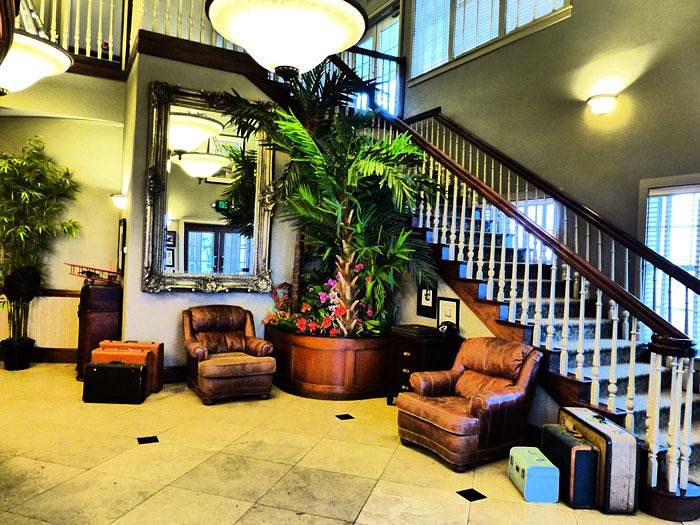This color photograph captures the interior of a brightly lit home, viewed from the perspective of someone standing near the front door. The room features a staircase with a wooden banister on the right side, leading upward from the bottom left corner of the image. Adjacent to the staircase is a white tile floor decorated with small black diamonds at the intersection of every four tiles. Positioned prominently in the corner near the staircase is a large potted plant with lush palm fronds and colorful red and pink flowers at its base. 

To the left of the plant, mounted on the wall, is a large mirror encased in an ornate silver frame. Below the mirror sits a well-worn brown leather armchair. Another similar leather armchair is set against the staircase, facing slightly towards the area between the staircase and the wall. Both armchairs exhibit signs of heavy use. 

Clustered below the mirror to the right of the armchair, and next to the other armchair by the staircase, are three suitcases, suggesting recent travel. The ambient lighting casts a warm yellow hue across the room, enhancing its cozy yet slightly cluttered atmosphere.